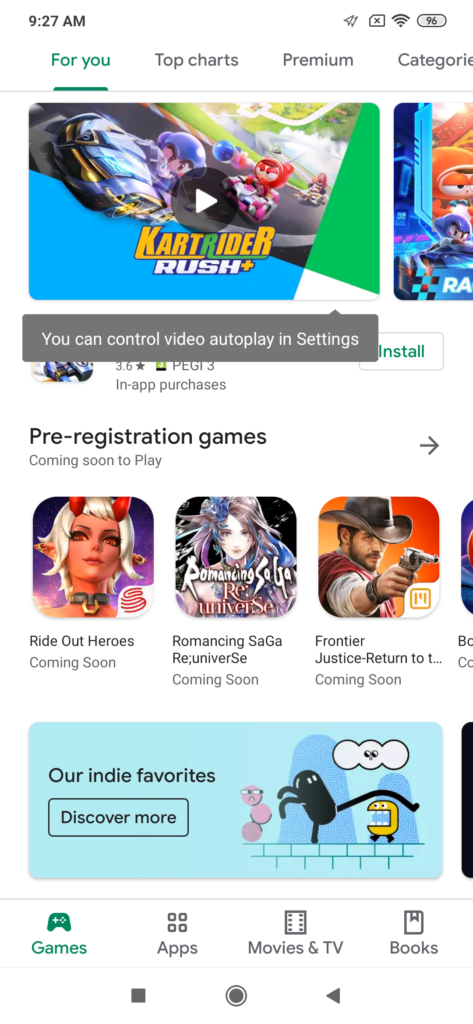Here is the cleaned-up and detailed caption for the image:

---

The image is a screenshot of a smartphone displaying the Google Play Store app. The status bar at the top of the screen shows it is 9:27 a.m., the battery level is at 96%, and both the Wi-Fi and network signals are strong. An unfamiliar icon is also present on the status bar.

Below the status bar, the "For You" section is highlighted, indicating it is currently active. Other tabs available include "Top charts," "Premium," and "Categories."

The main content features a clickable video thumbnail for the game "Kart Rider Rush," highlighted by a pop-up that reads, "You can control video autoplay in settings." Unfortunately, much of the game information is obscured by the pop-up. However, visible details indicate it has a PEGI 3 rating, in-app purchases, and an "Install" button.

Further down, the screen reveals a section for "Pre-registration games coming soon to play," indicated by a right-pointing arrow. Three game thumbnails are displayed: "Right Out Heroes," "Romancing Saga Reuniverse," and "Frontier Justice - Return 2," although some titles are partially obscured.

A whimsical cartoon image appears next, possibly showing a bean-shaped character interacting with other bizarre figures. This section is titled "Our Indie Favorites, discover more."

At the bottom of the screen, navigation tabs include "Games," "Apps," "Movies & TV," and "Books," with "Games" currently highlighted in green. The bottom-most row features typical Android navigation buttons: a square, a circle, and a triangle.

---